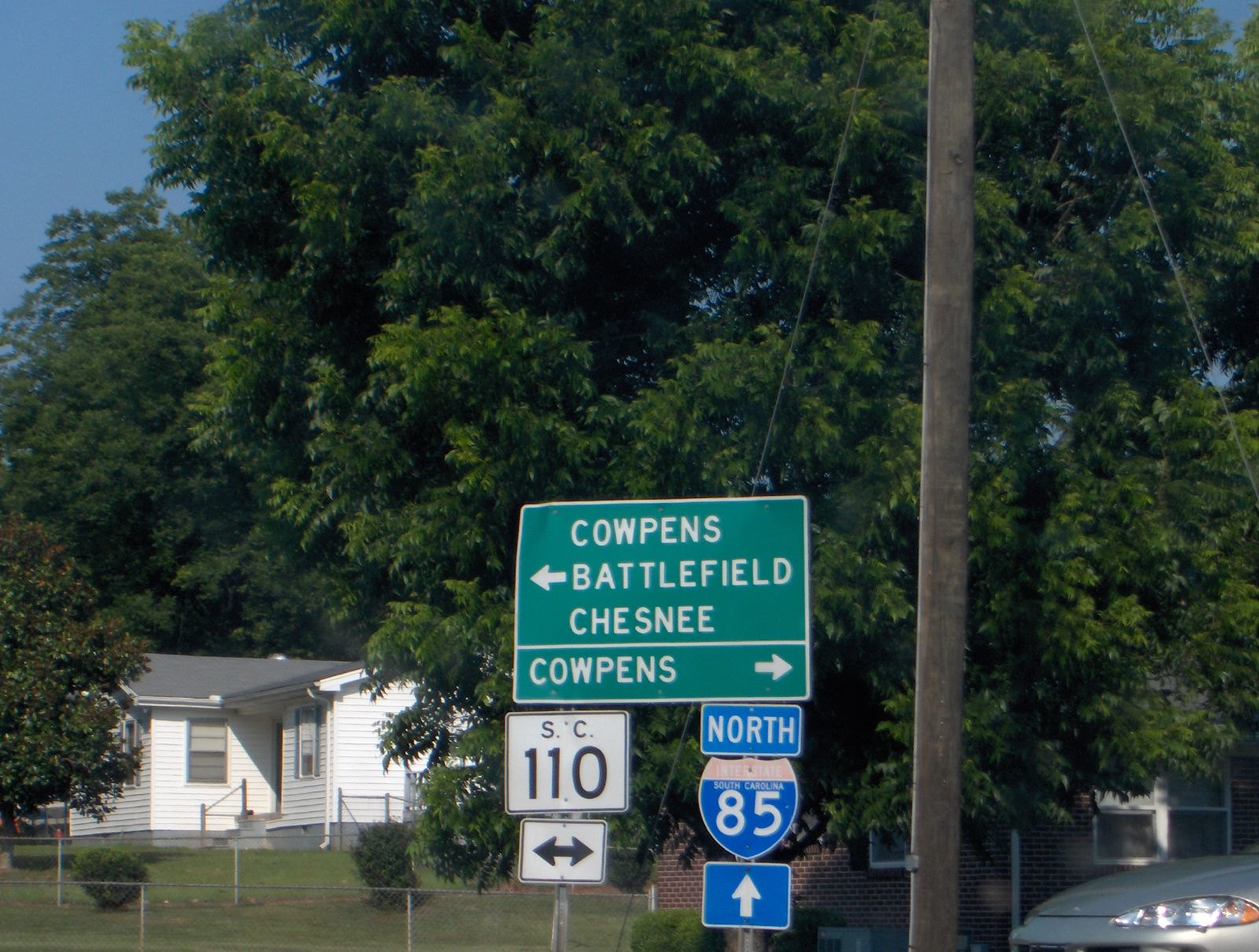This photograph captures a detailed streetscape featuring an array of traffic signs and suburban elements. Prominently displayed is a green directional sign with white lettering: an arrow pointing left reads “Cowpens Battlefield”, “Chesney,” and an arrow pointing right says “Cowpens.” Below this, a white sign for "SC-110" displays arrows pointing in both directions. Also included is a sign "North Interstate 85 South Carolina" with an upward arrow indicating the highway ahead. To the right of the signs, there is a silver car parked or stopped near a wooden electrical pole. The background showcases a modest brick house with a fence, and adjacent to it, a white house with slat-board siding and a gray roof. A lush tree with green leaves partially obscures the houses, and another tree is visible behind the white house, complementing the suburban atmosphere.